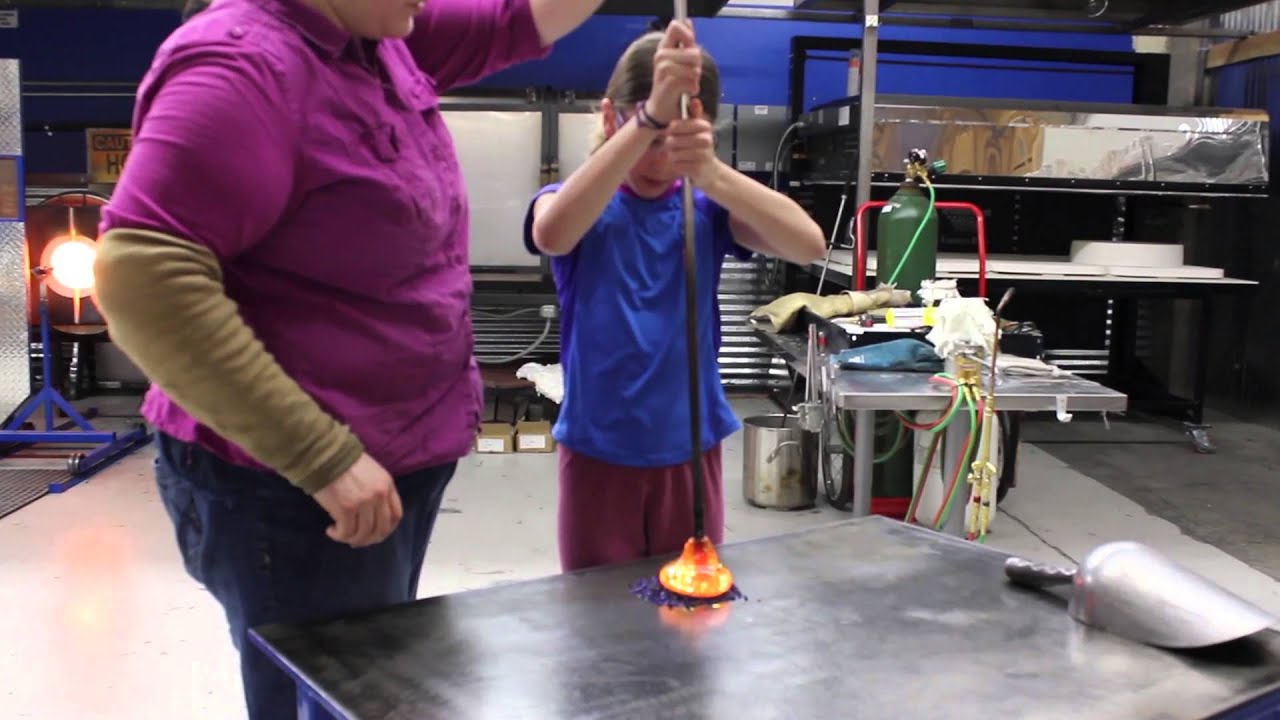In the image, a young girl, approximately eight years old, is engaged in an industrial setting, likely a machine shop or a lab specialized in glassblowing. She is standing in front of a stainless steel table, wearing a blue shirt and purple pants. In her hands, she holds a long pole with a red-hot, melted object at the end, which she appears to be shaping on the table. To her left, partially visible, is an adult instructor wearing a purple shirt with burn-resistant brown-green sleeves and dark pants, seemingly assisting her.

The background of the room features a blue wall and a cluttered table filled with various mechanical items. On the left-hand side, a glowing hot kiln is emitting bright light, indicative of a very high temperature, likely used for glassblowing. Behind the girl, a green canister with red lines is also noticeable, possibly related to the lab's equipment. The floor of the space is concrete, adding to the industrial atmosphere. On the right side of the image, there are more chrome-finished pieces of equipment and another metal device with cords extending from it. A small metal scooper rests in the lower right corner of the table. This scene encapsulates the intricate processes involved in working with heated materials within a well-equipped industrial lab.